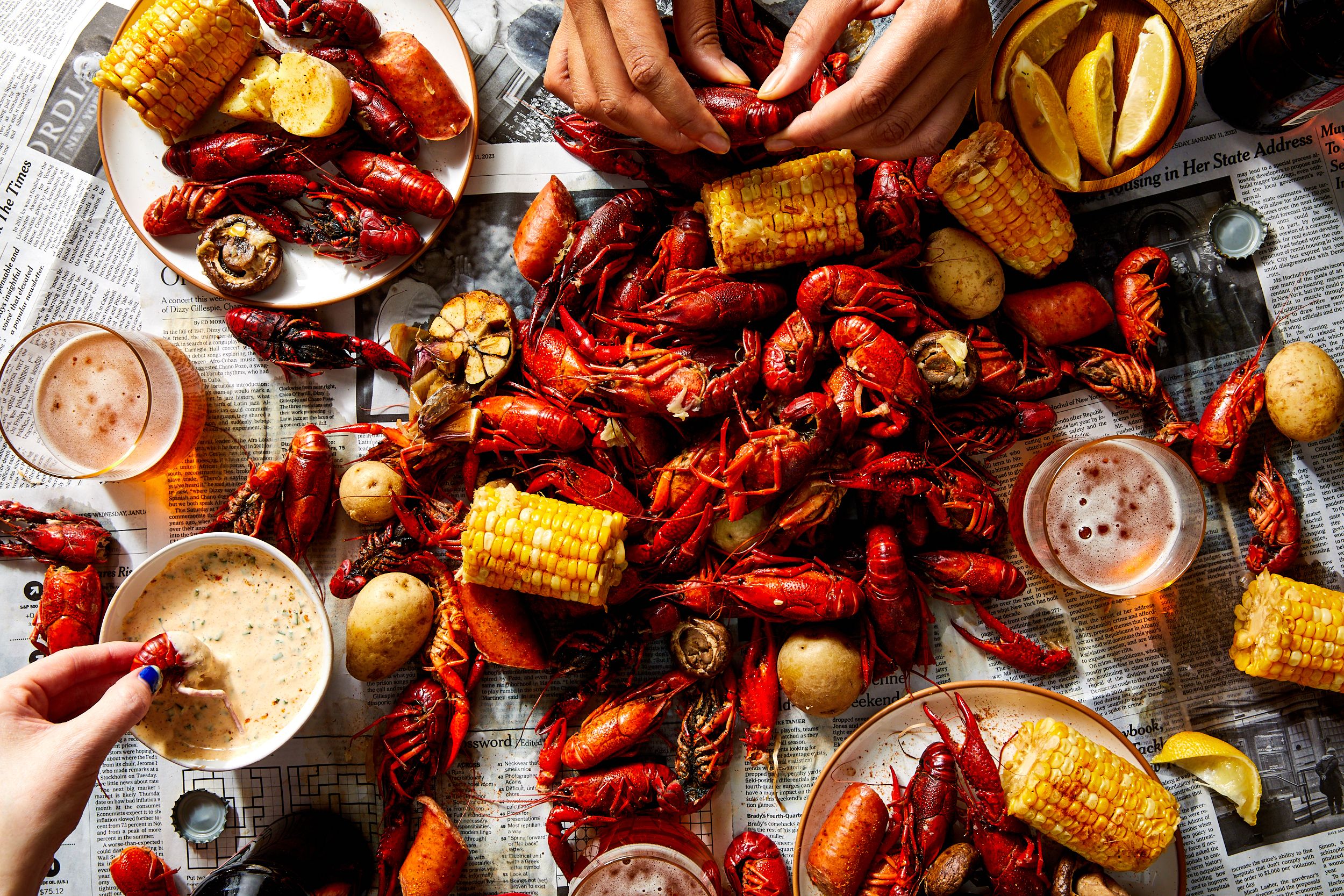This vibrant photograph captures a lively crawfish boil feast set on a table covered with newspaper. The centerpiece of the spread is a generous pot of freshly boiled crawfish, corn on the cob, baby potatoes, and savory sausage, all casually scattered across the paper. Surrounding this mouthwatering assortment are several plates, each neatly piled with portions of the same delectable fare, suggesting guests are well into enjoying the meal. Adding to the festive atmosphere are glasses of frothy beer standing at the ready, while small bowls of dipping sauce, presumably remoulade, offer a zesty complement to the seafood. Bright yellow lemon wedges are also scattered across the table, ready to be squeezed over the food for an extra burst of flavor. Amid the delicious chaos, a few hands reach in to either peel the crawfish or dip morsels into the sauces, highlighting the communal and interactive nature of this delightful Southern tradition.